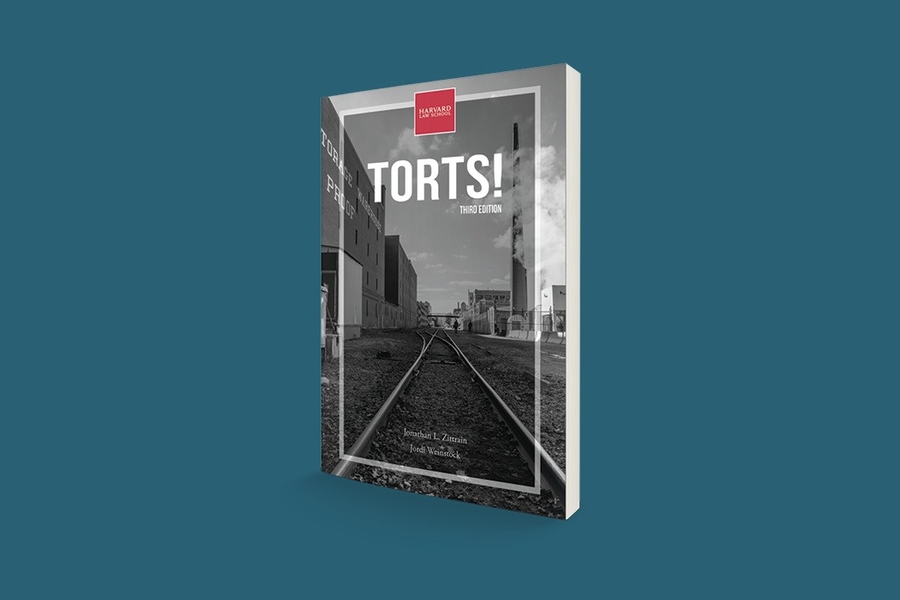This image showcases the cover of a book titled "Torts, 3rd Edition," prominently displayed against a blue-green background. The book, possibly published by Harvard Law School, features a striking black and white photograph of a railroad track leading into an industrial area or cityscape. A vivid red square positioned at the top of the cover contains the text "Harvard Law School." The authors, Jonathan L. Zittrain and Jordy D. Weinstock, are listed at the bottom. The book cover includes a white inner border framing the central image, adding to the presentation's clarity. The book itself appears to be roughly half an inch thick, with its spine angled away, showing rows of white pages.